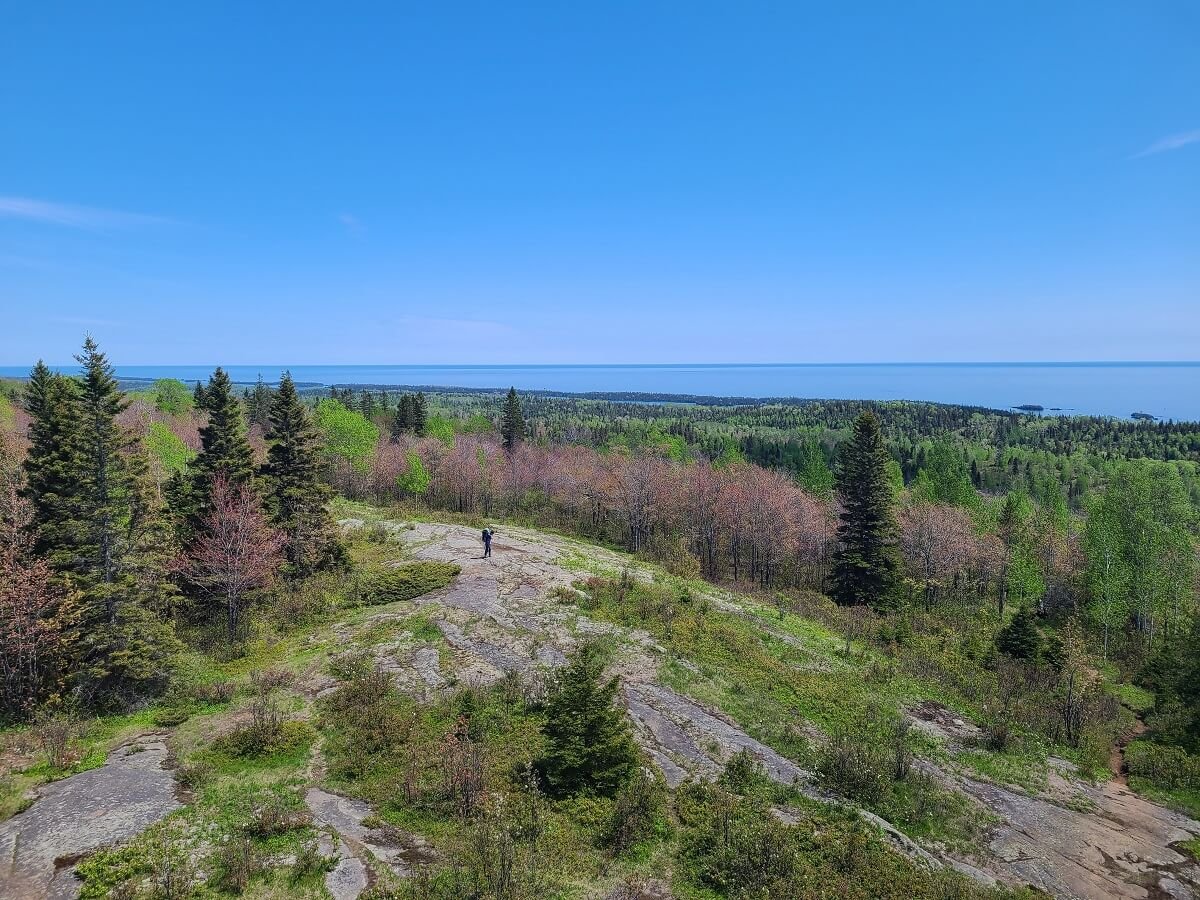An aerial view captures a breathtaking landscape from atop a rock cliff of a mountain, where patches of long-grown grass and trees thrive amidst the rocky formations. A lone person stands in the distance along the cliff's edge, gazing out over the sprawling scenery. Below, the scene transitions into an open forest dominated by a central sandstone trail flanked by evergreen trees and some shedding, colorless ones. This trail leads the eye through a densely wooded area toward a vast body of water. The foliage varies from green to bright burgundy hues, creating a striking contrast with the deep blue expanse of the ocean that stretches out to the horizon, where the sky, mostly clear with thin strips of clouds, seamlessly meets the water. The overall view provides a mesmerizing interaction between rugged natural elements and serene aquatic beauty.